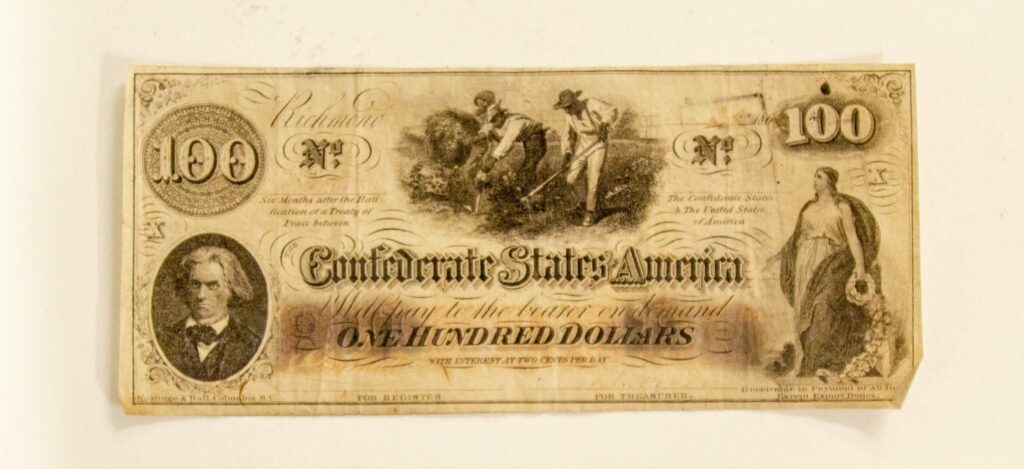This image is a close-up photograph of an antique $100 bill issued by the Confederate States of America, likely from the 1860s during the Civil War. The bill, which sits on a white countertop, has a vintage and sepia-toned appearance, suggesting its authenticity. In the center of the bill, prominently displayed, are the words "Confederate States of America $100." Both the top left and right corners feature circular emblems with "$100" inscribed.

On the left side of the bill is an oval portrait, possibly of Jefferson Davis, the President of the Confederacy, though there's no confirming text. To the right sits an image of a forlorn woman, intricately detailed in a Greek-inspired white gown with a flowing robe or shawl. The lower right corner of the bill is notably curled.

The central graphic captures a somber historical scene: multiple Black slaves working in a field, indicative of the manual labor and exploitation that supported the Confederate economy. They are depicted using hand tools like hoes, engaged in what appears to be agricultural work. The overall composition of the bill, from its detailed illustrations to its distinctive layout, encapsulates a complex, albeit troubling, piece of American history.